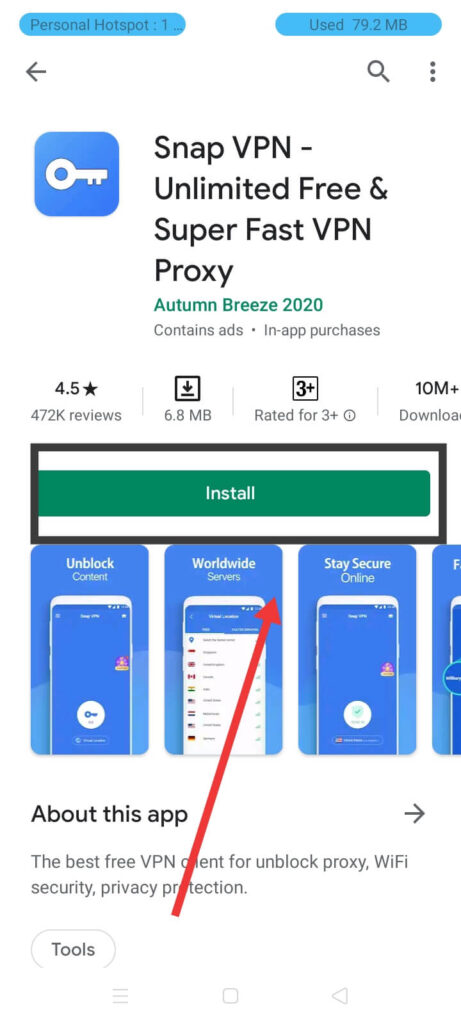In the upper left corner of the image, there is a long, thin, blue oval bearing the text "Personal Hotspot" in dark gray font, followed by a space, a colon, another space, the number "1," another space, and an ellipsis ("..."). Towards the right of this oval, a similar blue shape contains the text "Used 79.2MB." Below these ovals, the background transitions to white.

On the left side of the white background is a gray arrow pointing to the left, indicating navigation to a previous page. Towards the right of the arrow is a magnifying glass icon, slanted with the bottom towards the right and the top towards the left, signifying a search function. Adjacent to the magnifying glass, three vertical gray dots suggest the presence of a drop-down menu.

Moving further right, there is a rounded square app icon with a blue background displaying a white key oriented horizontally with the long part pointing to the right. Below the icon, the app name is written in black as "Snap VPN - Unlimited Free & Super Fast VPN Proxy." Directly beneath this, "Autumn Breeze 2020" is displayed in green, bold font of a smaller size. Below this, a light gray text indicates "Contains Ads • In-app purchases."

Further down, the app has garnered a 4.5-star rating based on 472,000 reviews. Next to this, a download symbol is present with the information that the app takes up 6.8 megabytes of space. To the right of these details, the app is noted as being rated for users aged three years and up. Finally, there is information that the app has been downloaded 10 million times.